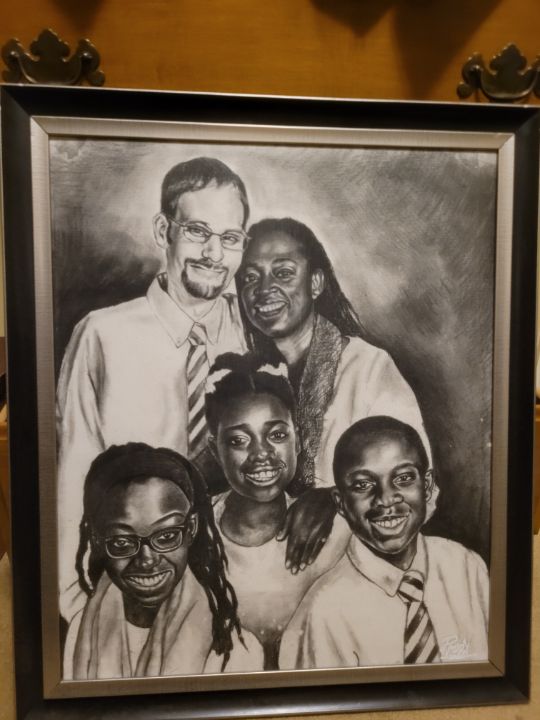A meticulously detailed black and white hand-drawn portrait of a multicultural family, framed in a square black and gold-trimmed frame. The portrait captures five family members: the father and mother stand behind their three children. The father, a white man with glasses, a mustache, a short goatee, and short hair, is dressed in a collared button-down shirt with a striped tie. The mother, a black woman with long hair flowing behind her neck, smiles warmly, wearing a shirt and scarf. She rests her hand on the shoulder of their middle child, a young girl. The two daughters, one with dreadlocks and the other with a bun adorned with a ribbon, sit or stand contentedly alongside their brother, who also dons a button-down shirt and striped tie. Each family member’s attire is rendered in shades of gray, emphasizing their light-colored clothing. Their facial features are intricately conveyed, capturing their smiles and expressions in fine detail. Behind them, a subtly drawn background suggests a light wooden drawer with small, riveted metal handles, enhancing the intimate, homey atmosphere of the portrait.